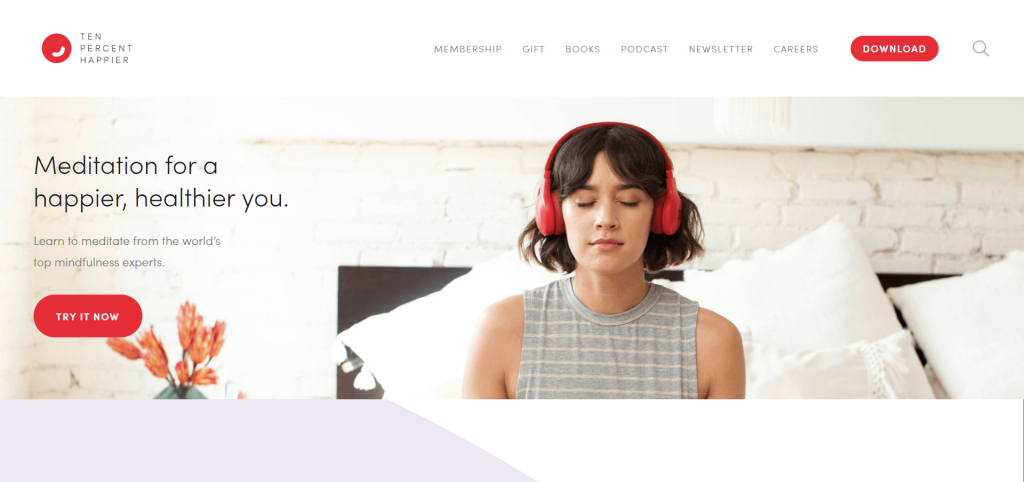In the image, a woman is seated in the center of a neatly-made bed, appearing to meditate with her eyes closed. She is wearing red headphones and a gray shirt, creating a serene and focused look. The backdrop is a white brick wall, adding a touch of minimalist comfort to the room. The bed has white pillows which complement the calming atmosphere.

In the upper left corner of the image, there is a logo for "10% Happier" featuring a red circle with a white line through it, suggesting this might be the brand or website’s name. The top of the page displays navigation tabs for Membership, Gift, Books, Podcast, Newsletter, and Careers. Additionally, a prominent red download button and a magnifying glass icon for search functionality are visible.

To the left of the woman, the text reads: "Meditation for a happier, healthier you. Learn to meditate from the world's top mindfulness experts." Below this message, there is a red button labeled "Try it now." The overall scene appears to be an advertisement or promotional content for a meditation program or application, offering a tranquil and inviting introduction to potential customers.